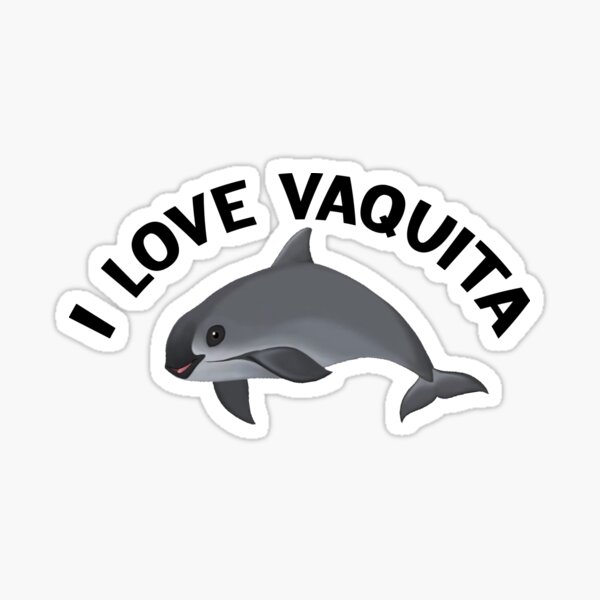This is an image of a sticker design composed of three separate stickers spelling out "I LOVE VAQUITA" in black, all-caps letters with a white outline, arranged in an arch above an animated vaquita. The vaquita, often mistaken for a dolphin, is illustrated in profile facing left, with anthropomorphic features that give it a smiling, human-like expression. The vaquita's body features a black nose and mouth area, black front flippers, and a predominantly dark gray body that fades to a lighter gray on the throat and belly. The design includes a white border around the entire composition, set against a solid off-white background, creating a clean and minimalist appearance. The vaquita's tail is down, and it is posed as if floating, unattached to any water, with its overall proportions realistic but facial features distinctly humanized.